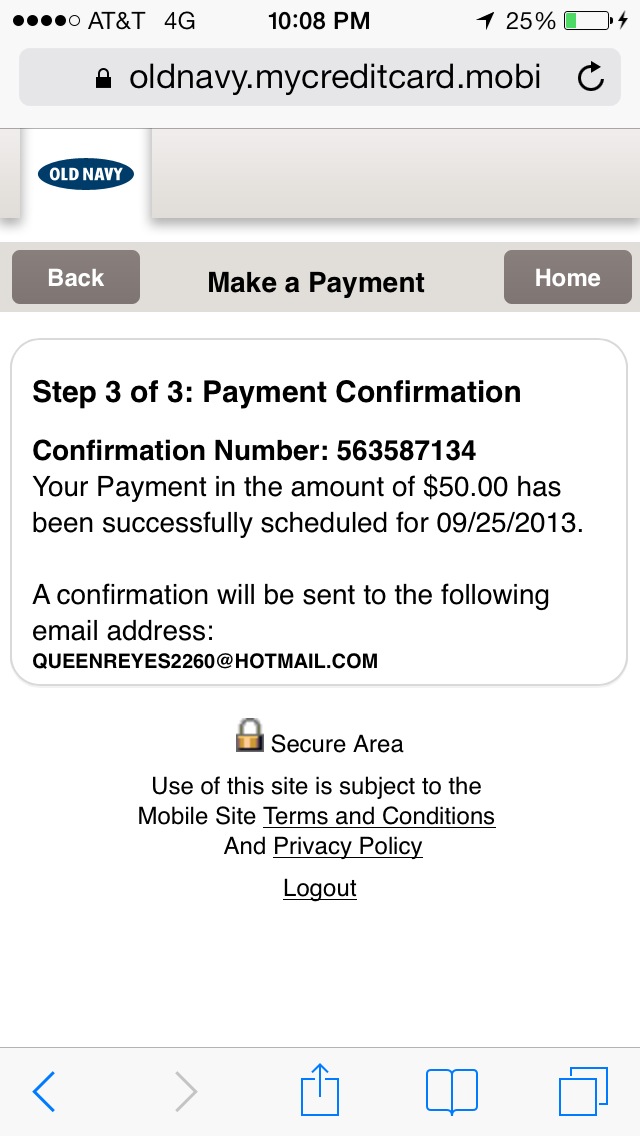The screenshot, taken from a cell phone in landscape mode, depicts a webpage in a light gray header. The status bar at the top shows 4 out of 5 service bars with AT&T 4G, the time 10:08 PM, location services icon, a battery icon displaying 25% and charging, all on the right end of the header. Below the header, the address bar reads "oldnavy.mycreditcard.mobi," indicating a secure site with a refresh button on the right. 

The main content begins with the Old Navy logo in a blue oval with white text. Underneath is a gray horizontal bar featuring a back button on the left, the text "make a payment" in the center, and a home button on the right, all in dark gray. Below this, a white box labeled "Step 3 of 3" contains the payment confirmation details: "Confirmation number 563587134. Your payment in the amount of $50 has been successfully scheduled for 09-25-2013. A confirmation will be sent to the email address quenreyes2260@hotmail.com." 

Further down, an icon of a padlock is accompanied by the words "secure area." It is followed by the disclaimer: "Use of this site is subject to the mobile site terms and conditions and privacy policy." The screen ends with an underlined "Log out" option. Along the bottom of the screen, there is a light gray border housing navigation icons: a blue back arrow, a gray forward arrow, a blue share icon, a blue bookmark icon, and a blue new page icon.